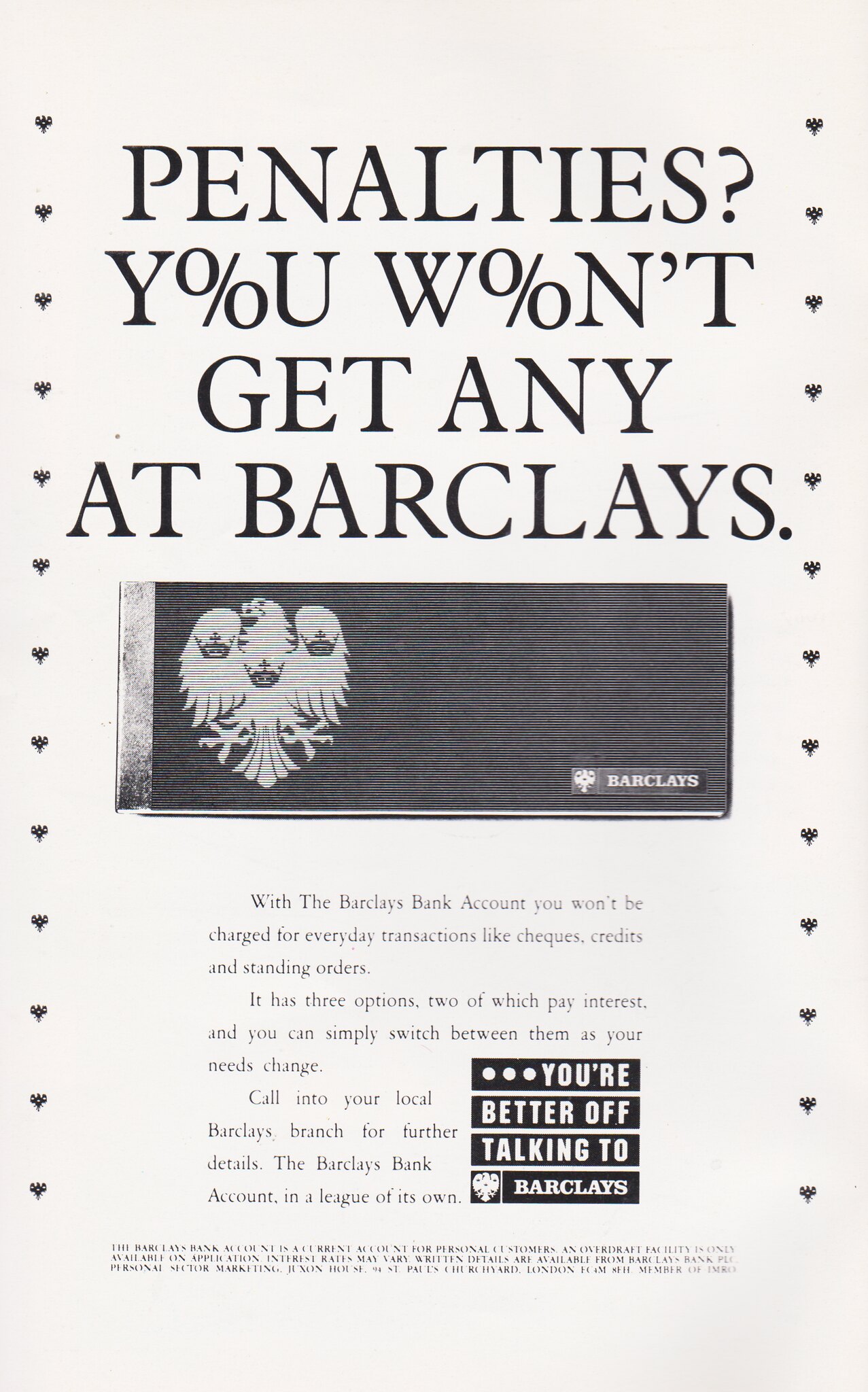This advertisement for a Barclays card, likely from an older era, features a predominantly monochromatic color scheme with whites, grays, and blacks, giving it a vintage look. At the top, bold black letters pose the question, "PENALTIES? YOU WON’T GET ANY AT BARCLAYS," creatively replacing the 'O's in "YOU" and "WON'T" with percentage signs. Below this text is the Barclays logo, depicted in black and white, showcasing an eagle with three crowns. The advertisement assures readers that with a Barclays bank account, there are no charges for everyday transactions such as checks, credits, and standing orders. It also mentions the flexibility of switching between three account options, two of which offer interest, to suit changing needs. The words, "You’re better off talking to Barclays," appear prominently at the bottom within a black banner, inviting potential customers to visit their local Barclays branch for further details. The overall layout features the main question and statement at the center top, the logo centrally placed, and additional descriptive text below, emphasizing the benefits of banking with Barclays.